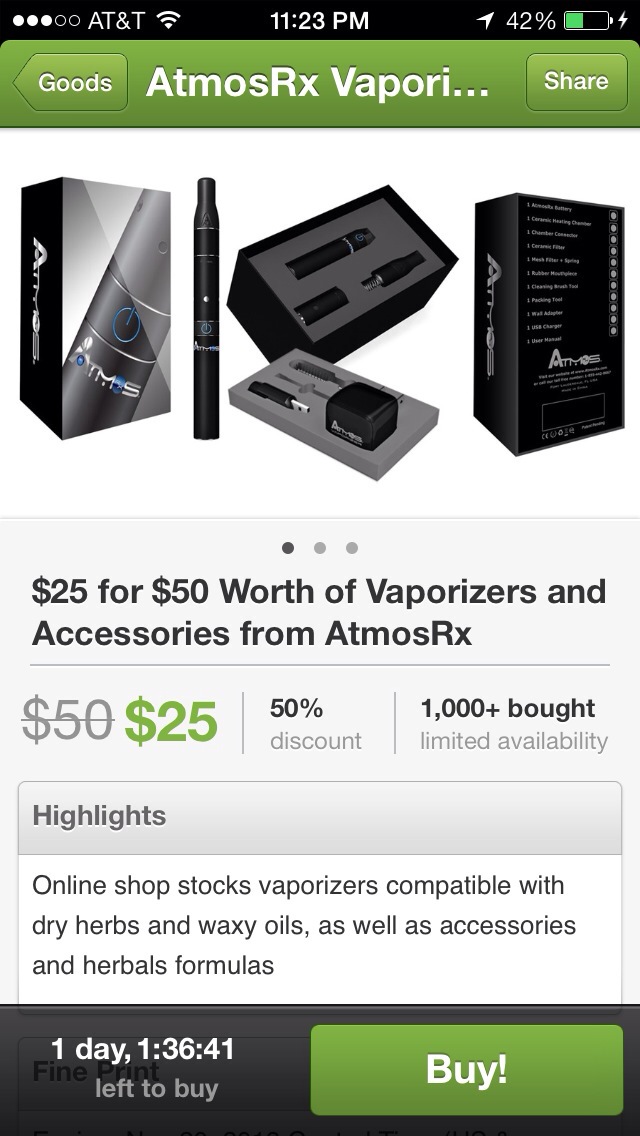This image depicts a detailed screenshot taken from an iOS device, specifically an online shopping app showing a promotional deal for Atmos RX vaporizers. The screenshot, occupying the entire frame, is marked by the device’s status bar at the top, indicating it’s 11:23 PM on an AT&T network with a battery life at 42%. Below this, the central focus is on an advertisement banner with an image showcasing a vaporizer and its accessories both in and out of its packaging.

In bold black lettering, the offer prominently states "$25 for $50 worth of vaporizers and accessories from Atmos RX," with the original $50 price crossed out and replaced by a green $25 mark, signaling a 50% discount. Additional text confirms "1000+ bought" and highlights the available stock of vaporizers compatible with dry herbs and waxy oils, along with accessories and herbal formulas. Below this, there’s a countdown timer indicating “1 day, 1 hour, 36 minutes and 41 seconds left to buy”.

At the bottom right corner is a big green buy button in white letters with an exclamation point, urging immediate action. The overall color scheme incorporates black, white, green, and gray elements, maintaining a clean and commercial aesthetic that clearly targets online shoppers looking for a deal on vaping products.